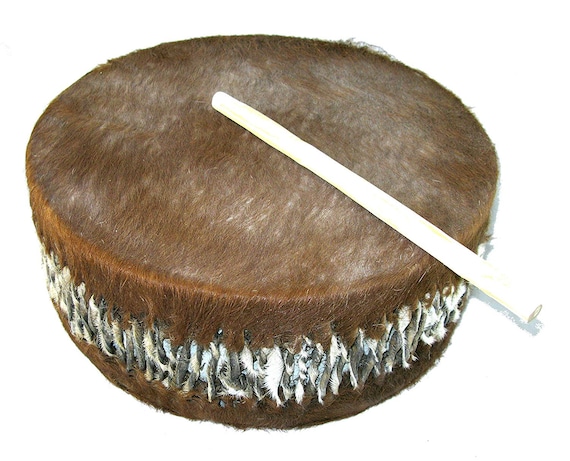This color photograph features a distinctive brown drum, likely crafted from animal hide. The drum, which is round but appears to be only a few inches tall, displays a rich gradient of brown from top to bottom. The top of the drum is covered in brown fur, indicating the use of animal hide, with lighter, whitish hide visible underneath. Resting on the top is a white drumstick, long and oval in shape, oriented horizontally from left to right. Around the middle section of the drum, amidst the darker brown hues, there are white feathers or feather-like materials integrated into the design, adding a contrasting element. The bottom of the drum mirrors the top with a continuation of the dark brown fur, completing the textured, natural look of the instrument.